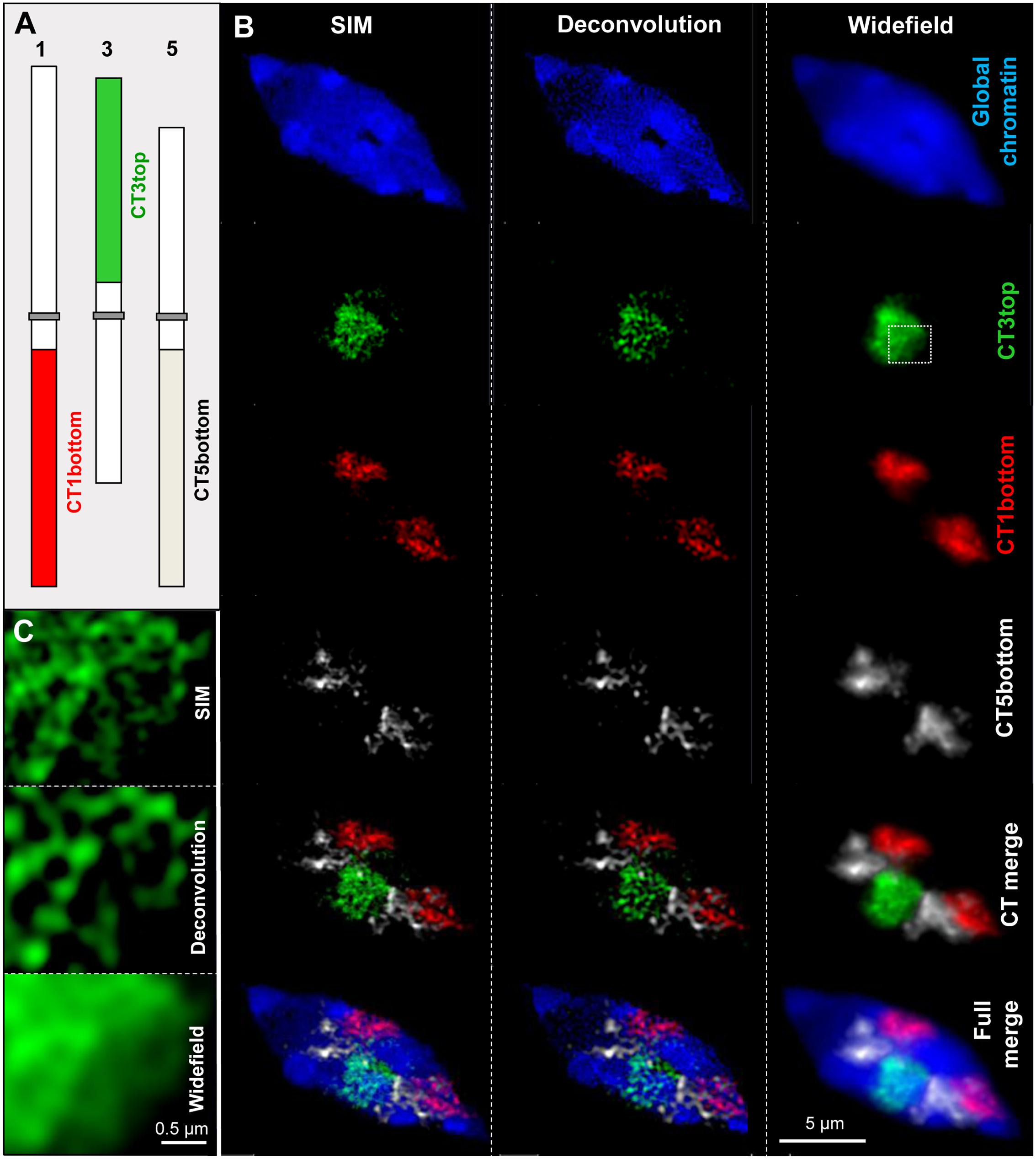This scientific diagram features three distinct columns labeled "Wide Field," "Deconvolution," and "SIM" from left to right. Each column showcases vibrant color smears in shades of blue, green, red, and occasionally multi-color blots. On the left side, there’s a vertical gray sidebar displaying three slider scales, accompanied by smaller, highly zoomed-in insets, likely images of leaves or tree structures. The corner text mentions terms such as "CT1 bottom," "CT5 bottom," and "CT3 top," suggesting specific scanning or imaging modes. Further annotations include "1, 2, 3, A," and "global chromatin," hinting at detailed labeling and segmentation within the diagram. The image appears to represent an intricate scientific study or visualization, possibly related to cellular structures or imaging techniques.